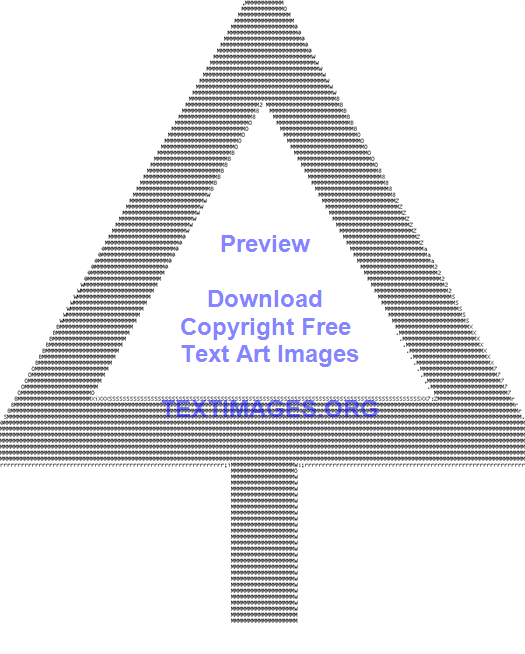The image appears to be a digitally created graphic featuring a tree-like shape designed with text. The primary shape resembles an equilateral triangle, symbolizing the tree's foliage, and a narrow vertical rectangle representing the tree trunk. Both elements are meticulously outlined with minuscule, repeating black symbols or letters, creating a thick and intricate border. The interior of the triangle is left as a solid white area, blending seamlessly with the flat white background of the image. Overlaying this design, semi-transparent blue text displays the words "Preview, Download, Copyright-Free, Text Art Images" centered vertically. Below this, in all caps, it reads "textimages.org," indicating the source of the image.